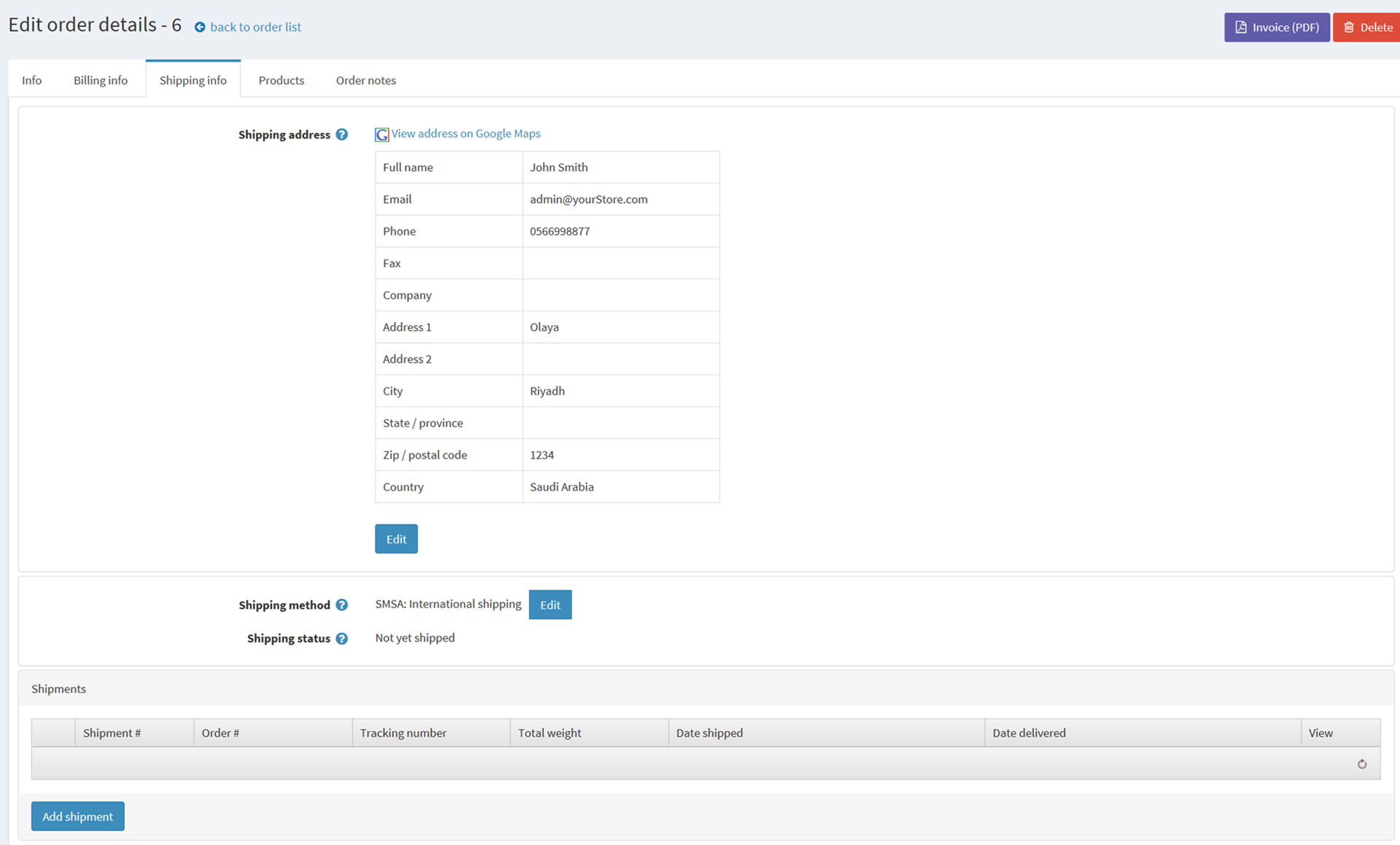The image showcases a detailed view of a website page, primarily focusing on an order management section. The page features a light blue header with two prominently placed buttons on the top right corner: "Invoiced PDF" in purple and "Delete" in red. Above these buttons, text reads "Edit Order Detail 6, Back to Order List."

Centered slightly towards the top left are multiple tabs labeled: "Info," "Billing Info," "Shipping Info," "Products," and "Order Notes." Positioned in the center of the page is the Shipping Address section, accompanied by a blue hyperlink text "View on Google Maps," which redirects to Google Maps.

The Shipping Address form includes fields with the following details:
- Full Name: John Smith
- Email: admin@etios.com
- Phone: 05666998877
- Fax: (Empty)
- Company: (Empty)
- Address 1: Olaya
- Address 2: (Empty)
- City: Riyadh
- State or Province: (Empty)
- Postal Code: 1234
- Country: Saudi Arabia

Next to this form is a blue "Edit" button.

Below the Shipping Address section, the page displays the "Shipping Method" as SMSA International Shipping, accompanied by another blue "Edit" button. There is a "Shipping Status" indicated as "Not Yet Shipped."

At the bottom section of the page, there is a table listing shipment details with columns titled: "Shipment," "Order Number," "Checking Number," "Total Weight," "Date Shipped," "Delivery," and "View." On the bottom left, a blue button labeled "Add Shipment" is visible.